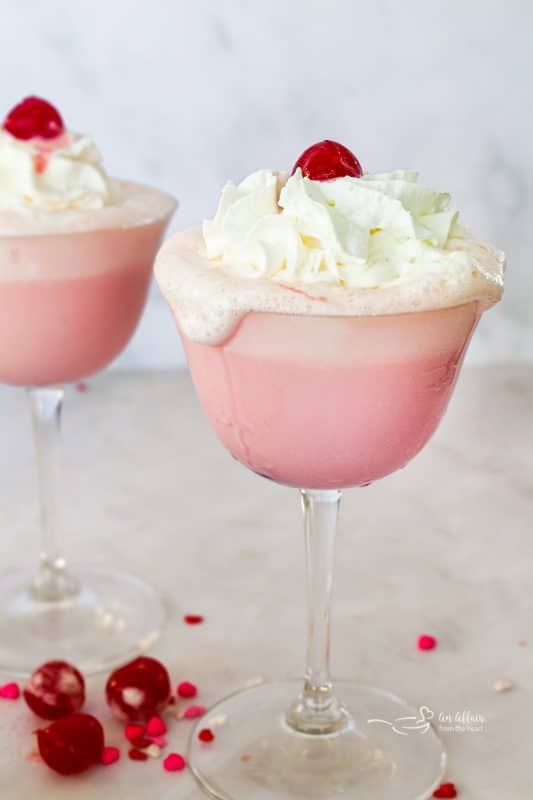The vertically rectangular, full-color photograph captures a close-up, indoor scene featuring a meticulously staged dessert presentation. Set against a nondescript white background, possibly a tarp or wall, and atop a light gray marble countertop, sit two identical, long-stemmed clear glasses, resembling large wine glasses. Each glass is filled with a pinkish creamy dessert, likely a strawberry daiquiri, that transitions into a lighter pink froth near the top. This frothy layer bubbles slightly over the edges of the glasses. At the center of the dessert sits a generous dollop of whipped cream crowned with a cherry. The foreground glass has whipped cream oozing and dripping down its side. On the countertop between the glasses lie three cherries and scattered dark red, pink, and white candy flakes, adding additional splashes of color to the elegant composition.